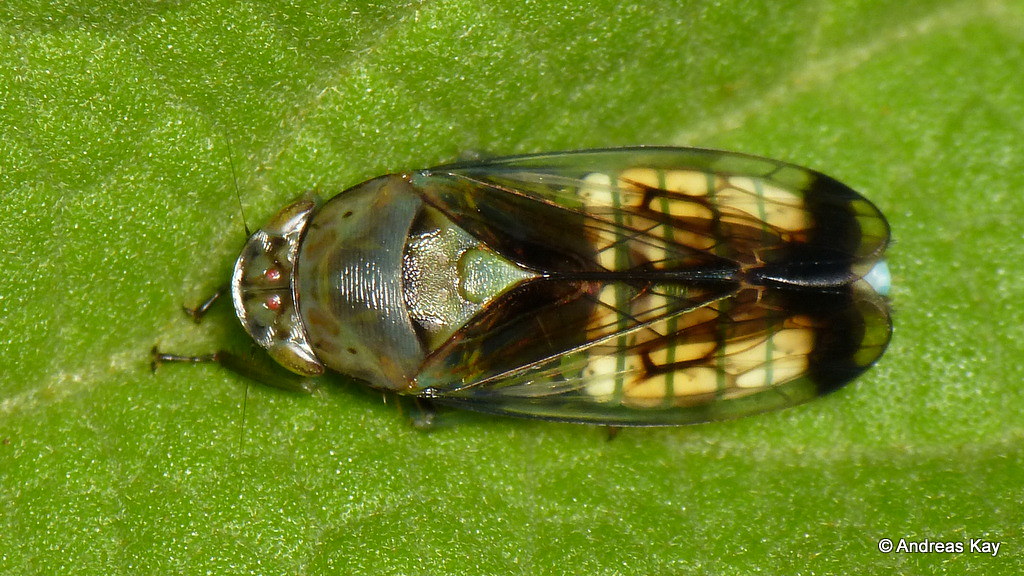This close-up image captures an insect, possibly a moth or cicada, resting on what appears to be a green leaf. The image is so detailed that you can see the intricate features of the bug. The insect is facing to the left, with delicate, transparent wings that showcase spots of black, brown, and green. There's a reflection of white and yellow light on these mostly see-through wings. The bug's body is visible beneath the wings, featuring a white-tan color with green stripes running across its abdomen. The thorax area is shiny, and its head is rounded, displaying slight antennae and little feet sticking out. At the bottom right of the image, a copyright symbol followed by the name "Andreas K" appears in white text. The green, shiny surface the bug rests on adds a vibrant background to this detailed close-up.